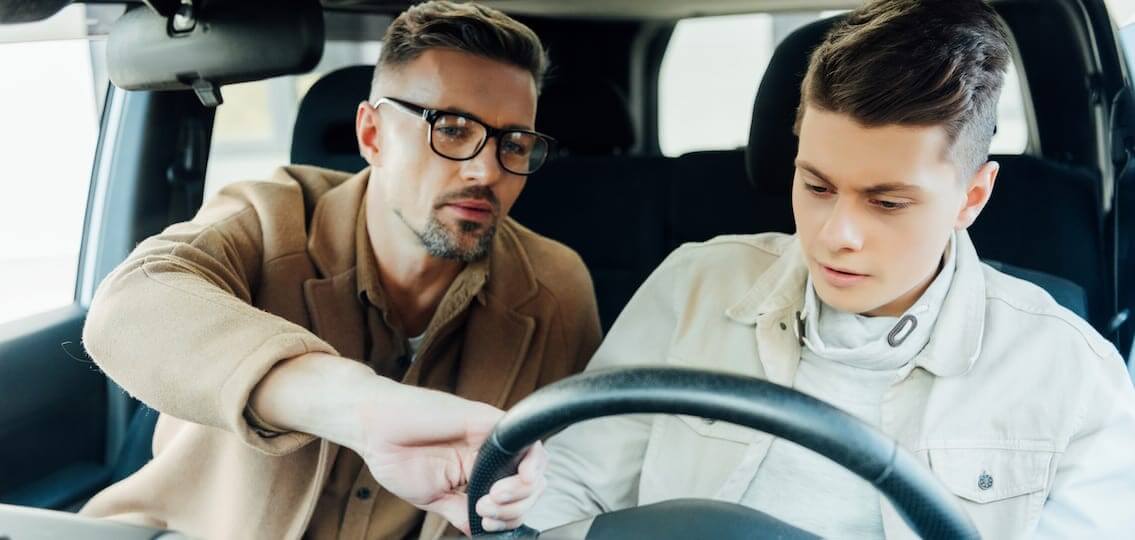The image depicts a heartfelt moment inside a car where a middle-aged dad is teaching his son how to drive. The scene is viewed through the windshield from an angle that captures both the father and son in the front seats. The father, wearing a light brown coat, black-rimmed glasses, and sporting a goatee, is seated in the passenger seat. He is intently leaning over with his right hand on the steering wheel, guiding his son. The son, clad in an off-white flannel or sweatshirt, has short brown hair and is deeply focused on the steering column. The car interior is black, and light filters through the side and back windows, creating a gentle illumination in the background. The concentrated expressions on their faces underscore the significance of this teaching moment.